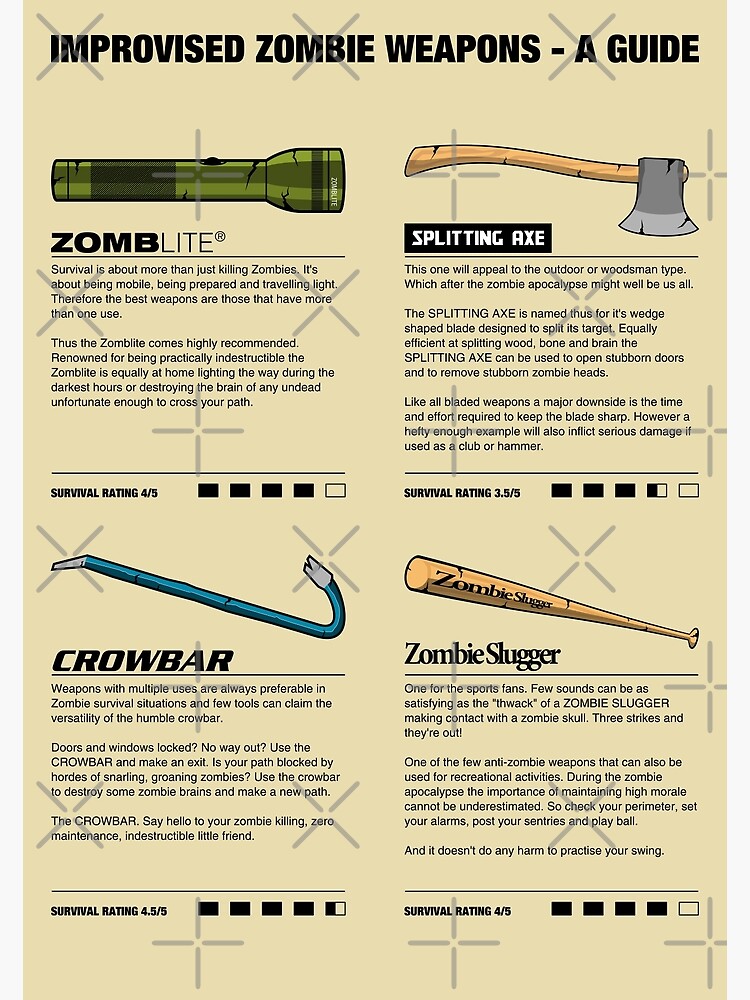This advertisement poster, designed on an 11 by 17 tan eggshell background, promotes "Improvised Zombie Weapons: A Guide." The layout is divided into four quadrants, each showcasing a different weapon with detailed descriptions and survival ratings below. 

- **ZOMB Light**: Positioned in the upper left, this olive green flashlight is identified with bold caps "ZOMB light" in thinner lettering. Its use is detailed in two to three paragraphs below, and it boasts a survival rating of 4.5 out of 5.
  
- **Splitting Axe**: To the upper right is a standard axe with a wooden handle and a silver blade, named the "Splitting Axe." Accompanied by a description, it has a lower survival rating of 3.5 out of 5.

- **Crowbar**: In the bottom left, there's a blue and silver-tipped crowbar labeled "Crowbar," also detailed with usage information, and it shares the high survival rating of 4.5 out of 5.

- **Zombie Slugger**: Lastly, the bottom right features a standard wooden baseball bat called the "Zombie Slugger." This weapon, with its description, is rated 4 out of 5 in survival effectiveness.

At the bottom, each weapon's rating is presented with black boxes checked off out of a possible five, reinforcing their utility in a survival scenario.